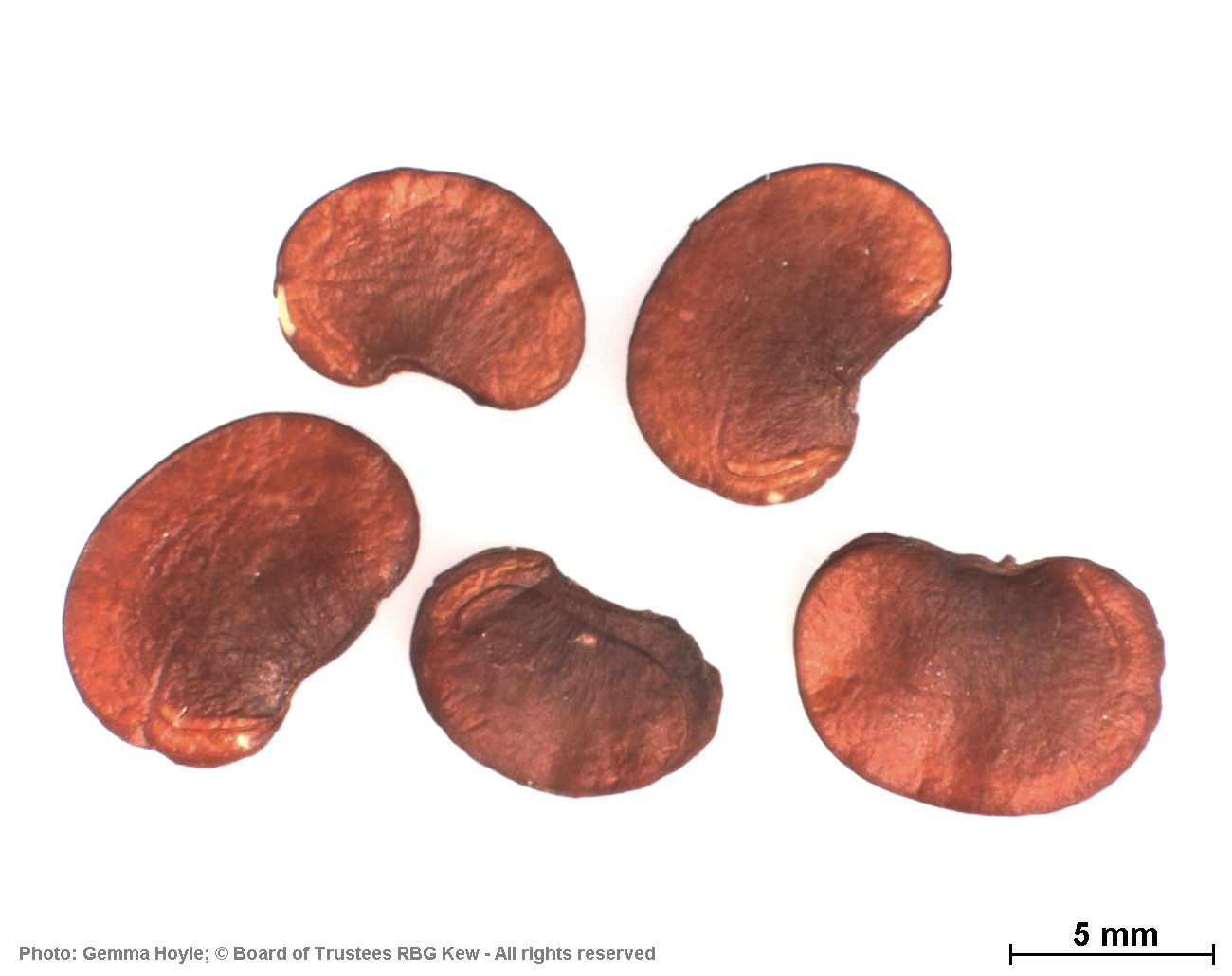The image features five brown, kidney-shaped seeds arranged against a white background. The seeds exhibit a gradient coloring, with darker brown in the middle and lighter brown towards the edges. There are two seeds in the upper row and three in the lower row, with the smallest seed positioned at the lower center. Some seeds have minor surface scrapes, revealing a lighter interior. At the bottom left corner, black text reads, "Photo: Gemma Hoyle. Copyright Board of Trustees RBGQ. All Rights Reserved." The bottom right corner includes a horizontal black line labeled "5 MM," serving as a scale to indicate the seeds' sizes, which are around 5 millimeters.